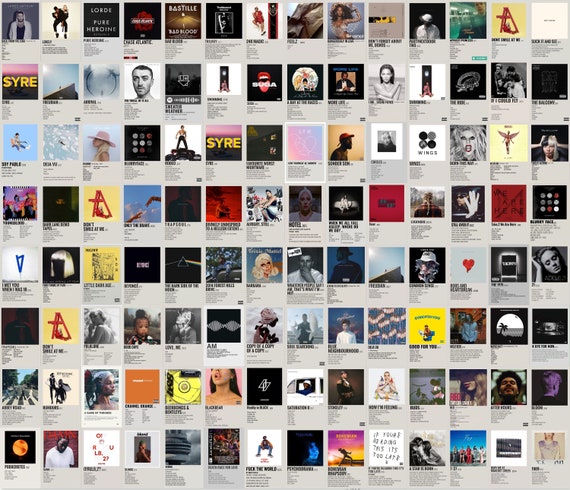This detailed and vibrant poster presents a comprehensive collection of album covers, with each thumbnail meticulously displaying the album artwork along with details about the album, the artist, and the producers. The poster features current albums from prominent artists such as Lorde, House Fuse, Heroines, Bastille, Beyoncé, Sam Smith, Sire, Lady Gaga, Kanye West, Adele, and in the bottom right corner, Taylor Swift's '1989'. Set against a white background, the array includes around a hundred diverse images, ranging from album covers to additional graphics like a rose, a triangle, and several faces of different ethnicities. Notably, the name 'S-Y-R-E' appears twice in bold yellow on a pink background. This square poster is not just an assembly of vibrant images but a colorful display of musical memorabilia, bringing a lively and eclectic mix of contemporary music right to the viewer's wall.